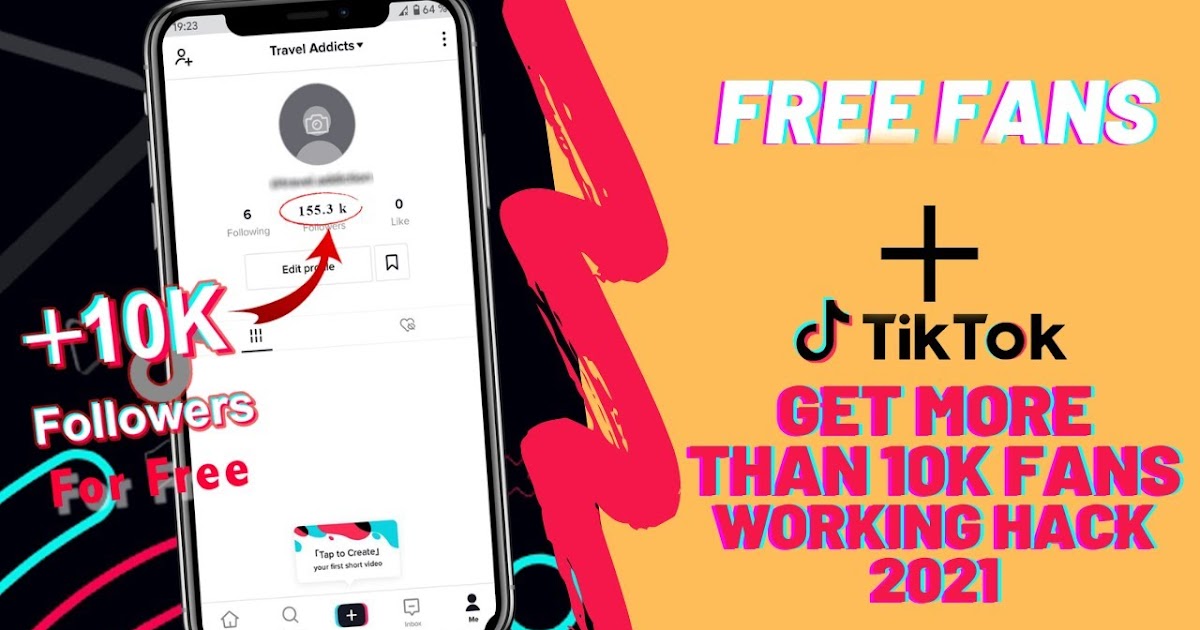The image is a colorful, landscape-oriented advertisement for TikTok, featuring a vibrant, eye-catching design. On the left-hand side, there is a smartphone display showing "153.3K Followers" with an arrow pointing towards it, captioned "Plus 10,000 followers for free." This suggests that users can buy or gain followers, which raises ethical concerns about the practice. The background on this side is predominantly black, adorned with playful, squiggly, and zigzag colored lines that resemble hand-drawn marker strokes, adding a lively and dynamic feel to the advertisement.

On the right-hand side, the background shifts to a bright yellow canvas. Large, bold white text reads: "FREE FANS + TikTok." Below this, in all caps, the following text is displayed in striking pink lettering with a subtle blue shadow, giving it a 3D effect: "GET MORE THAN 10,000 FANS WORKING HACK 2021." The TikTok brand logo is prominently featured in black, emphasizing the platform's association with the offer. The combination of vivid colors and bold typography aims to draw immediate attention and convey a sense of urgency and excitement for the viewer.